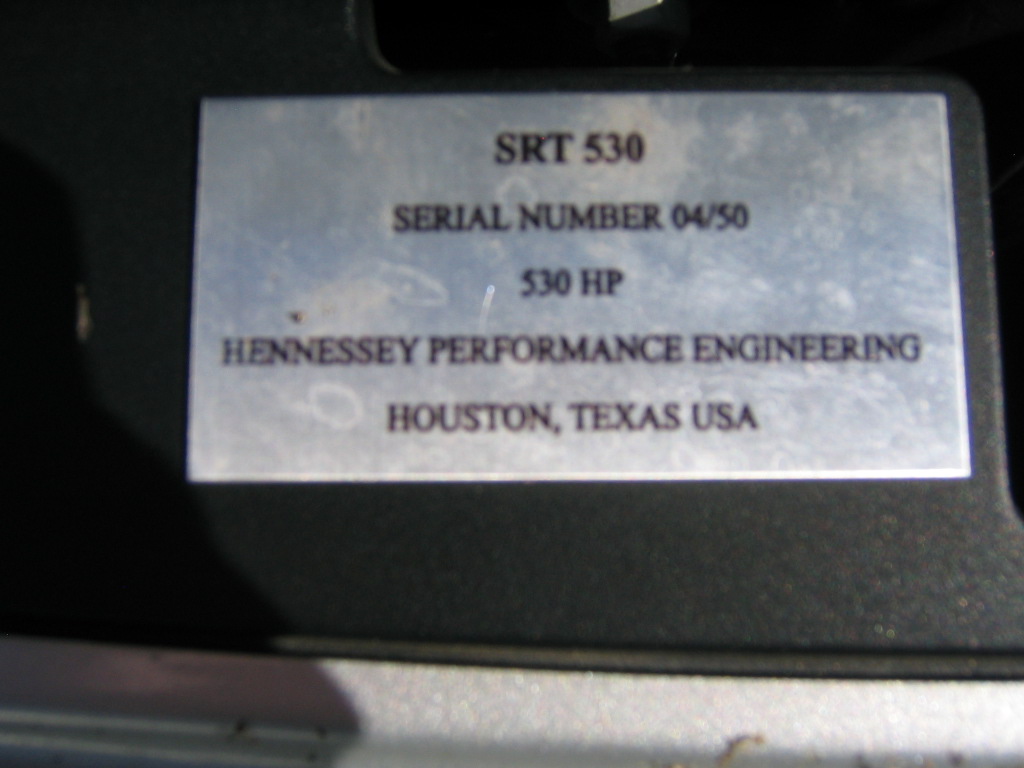This is a color photograph capturing a close-up view of a silver plaque mounted on a black surface. The image is slightly blurry, yet you can discern an almost yellowish, slightly golden reflection on the lower left edge where the surface is in shadow. The silver plaque, featuring a variety of silver hues, exhibits some minor wear, including round scratches particularly noticeable towards the left side. Inscribed in black text, the plaque reads: "SRT 530, Serial Number 0450, 530 HP, Hennessey Performance Engineering, Houston, Texas, USA." At the bottom, there is a silver band, with the left-hand bottom corner cast in shadow. Additionally, a small, rectangular grey shadow is visible at the top of the image, suggesting the presence of some kind of computer or electronic equipment just off-frame.